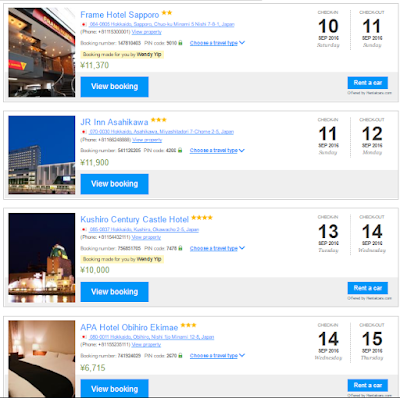The image depicts a section of a booking website focused on hotel reservations in Sapporo. Though the homepage lacks a title, it prominently features the name "Frame Hotel Sapporo" at the top. This specific section appears designed for travel planning and includes four distinct hotel booking options, each accompanied by images and details.

1. **Frame Hotel Sapporo:** The featured image showcases the exterior of the hotel. A blue box is visible, indicating an option to view the booking details. Alongside the image, the price is displayed, although the text is small and difficult to read. Additional details include dates marked with the numbers "10" and "11" and a blue box beneath these numbers stating "rent a car."

2. **JR Inn Sapporo:** This option presents an image of the hotel’s exterior, characterized by its attractive architecture. The option to view the booking is again available. The relevant dates for this hotel are labeled as "11" and "12." However, this segment does not include a car rental option.

3. **Crucio Century Castle Hotel:** The image here captures a stunning nighttime view of the hotel, fully illuminated. Booking details can be accessed via the "view booking" link, with the dates "13" and "14" highlighted. Additionally, beneath these dates, there is an option to "rent a car."

4. **APA Hotel Chiro Akimo:** The provided image illustrates the exterior of this hotel, with the caption including a "view booking" option for the dates "14" and "15." This hotel also offers a "rent a car" option.

Overall, this section of the website serves as an itinerary planner for hotel stays between the 10th and the 15th, offering varied accommodation options in Sapporo, with some including car rental services.